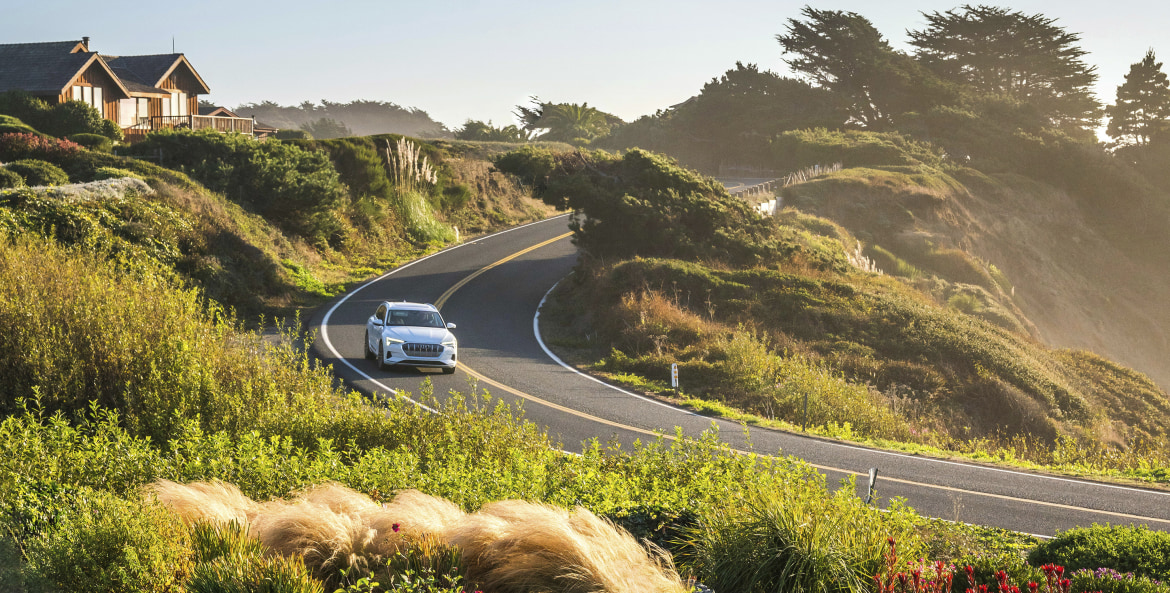A blue car, possibly electric, is shown driving from left to right on a curved, two-lane country road that slopes downward. The road is bordered by tall, green, and some brown grasses, with blooming feathery plants leaning due to strong winds. On the left side, a brick house with white windows and a black roof sits atop a hill with a steep drop to the road. Below the road, on the right side, there’s a very steep drop-off, hinting at a canyon or cliff face. In the background, a pale blue sky contrasts with dust or smoke rising from the canyon. The hillside is dotted with large trees, one of which has fallen and leans dangerously over the road, while the house’s area includes ornamental grasses mistaken for a creature. A small deck is visible on the house's side, and the scenery is completed with various shrubs and flowers adding color to the landscape.